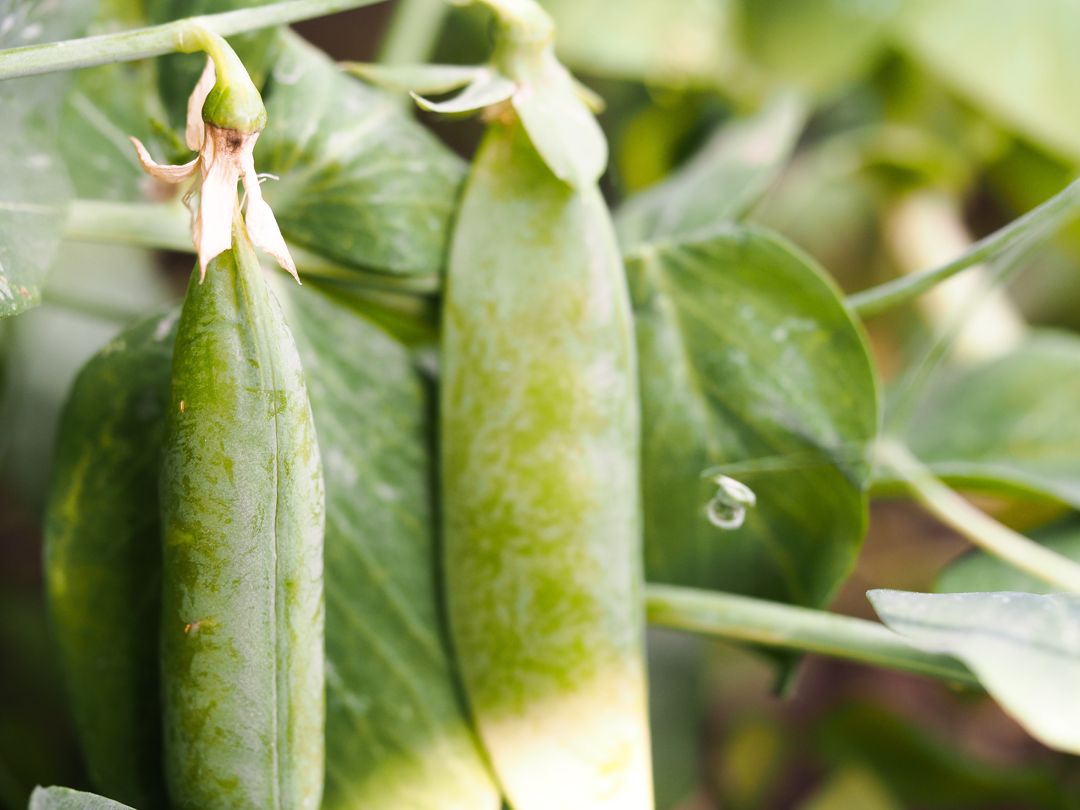This detailed close-up photograph captures a sunlit pea plant outdoors during the daytime. The image focuses on a green bean pod located on the left side, connected to a light green stem adorned with various dried brown leaves. The pod features a darker green indentation running along its center, signifying where it could be opened. The background and edges are heavily blurred, intensifying the focus on the central elements of the image. A larger, thicker green stem traverses the top left corner of the photograph, possibly indicating the main support of the plant. The surrounding green leaves, which are long and vertically aligned, are slightly out of focus and speckled with lighter green or whitish spots. A small, dried-out flower is present at the top of some leaves, adding to the natural texture of the scene. Overall, the photograph underscores the intricate details and textures of the pea plant captured in a garden setting.